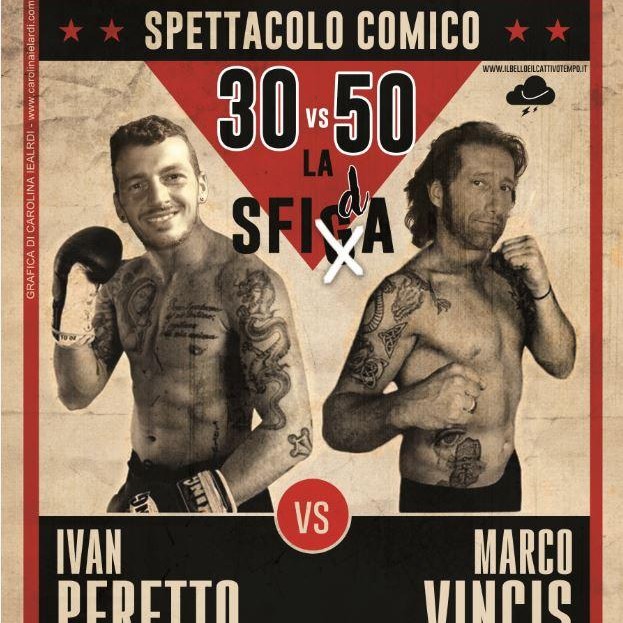The image is a detailed and striking newspaper clipping or an old poster advertising a boxing match. The background at the top is a solid black rectangular box, centered with the title "Spettacolo Kamiko" flanked by two red stars on each side. Below the title is a prominent red upside-down triangle featuring the numbers "30 versus 50" in large black digits outlined in white. Under this, there is the word "La Sfiga" with the 'G' crossed out and replaced with a lowercase 'D', transforming it to "La Sfida".

The focal point of the image features two male boxers, both heavily tattooed and bare-chested with dark trunks, their legs cropped out of the frame. To the left stands a short-haired man sporting a thin mustache and beard, complete with an earring in his left ear. His right arm is raised, showcasing a black boxing glove with a white inner section, while his left arm rests across his waist. On the right is another boxer with shoulder-length, slightly curly brown hair and a similar thin mustache and beard. This man, lacking gloves, has his left fist raised toward his chin and his right fist near his ribcage. 

Between the two fighters is a red circle with a white outline bearing the letters "V-S" in white. Their names are prominently displayed in large white letters; "Ivan Pareto" on the bottom left and "Marco Vincis" on the bottom right. The overall image includes distinct red accents against primarily black and white details, creating a stark and dramatic contrast that heightens the intensity of the fighters' stances.